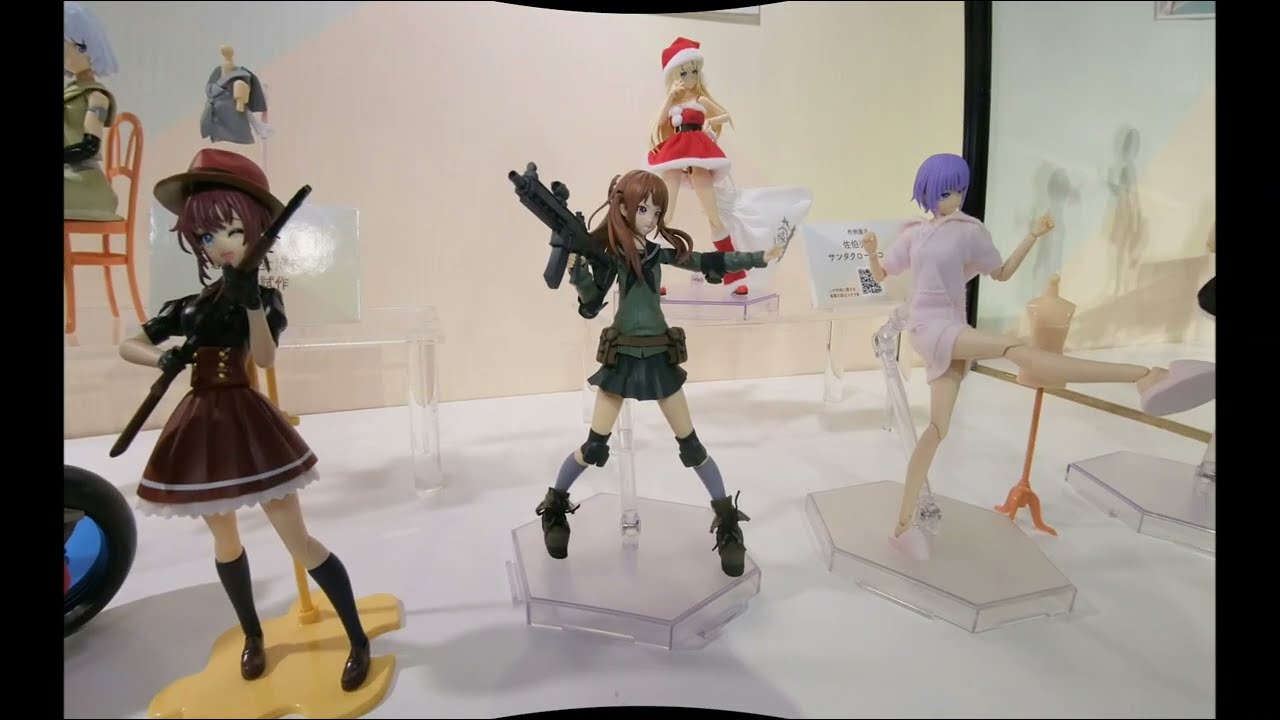The image showcases a collection of five to six slender, anime-inspired female action figures displayed on plastic pedestals within a white space. Each figure is adorned in distinct, elaborate outfits, suggesting a blend of cosplay and military themes. Notably, one figure in the back sports a provocative Santa Claus ensemble with a very short skirt and a striking pose. On the far left, another figure, only partially visible from the side, has light blue hair and is seated in an orange chair. In the forefront, a figure dressed in a brown short dress with knee-high black boots and a cowboy hat brandishes a small weapon. To her right stands a figure in a military-inspired green dress and combat boots, wielding an automatic weapon with arms outstretched. Finally, to her right, a figure in a pink dress with blue hair strikes a dynamic karate kick pose. Collectively, these figures create a vibrant and dynamic display, reflecting elements of anime and action genres.